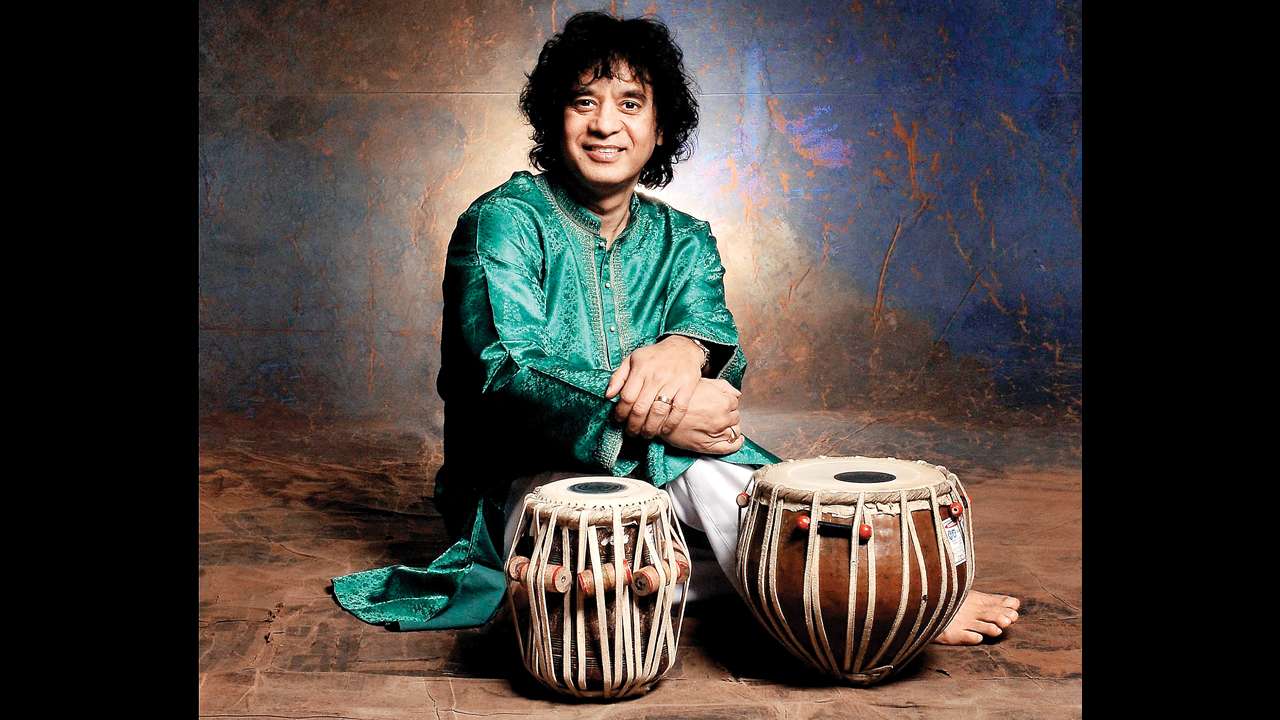In this vibrant photograph, celebrated Indian musician Zakir Hussain is captured sitting on the floor, emanating a sense of regal elegance in his traditional attire—a long green outfit paired with white pajamas, effortlessly blending luxury with cultural significance. His curly black hair frames his smiling face as he looks directly at the camera, exuding warmth and charisma. In front of him, two tablas—a traditional Indian percussion instrument characterized by their cylindrical shape and the distinctive black circle at the center of the drum skin—are positioned. The tablas feature a dark brown or black body adorned with a white fabric strip that could be leather, and the tops are lighter brown where the drum is struck. Zakir Hussain's hands are gracefully crossed, wearing a ring on one finger, showcasing his relaxed yet poised demeanor. The backdrop is a bit abstract with bluish-brown walls and a brown floor, adding to the colorful and artistic ambiance of the setting, which is undoubtedly steeped in musical tradition. Black rectangular frames on either side of the photograph add an additional layer of composition, enhancing the overall aesthetic.